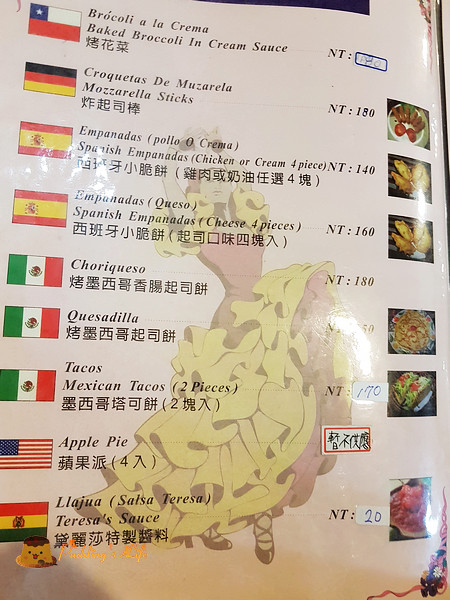The photograph showcases a vivid restaurant menu set against a pristine white background. The menu's glossy finish suggests it is either laminated or printed on shiny paper. Though the edges and top of the menu are not visible due to cropping, the centerpiece of the page remains unmistakable – a delicate, lightly colored illustration of a woman immersed in a flamenco dance. Her outfit is festive, featuring a red bodice with ruffled yellow sleeves and a striking skirt in red and yellow layers. Black strappy shoes complete her attire, and she exudes grace with her hands poised above her head.

Running along the left edge of the menu, a row of nine national flags hints at the diverse international cuisines offered. Adjacent to them, the next column lists the names of various dishes, each presented in both English and an Asian script, catering to a broader audience. Moving rightward, the subsequent column displays the prices. Notably, some prices have been updated with handwritten stickers, indicating new prices. Concluding the layout, the far-right column features colorful square photographs of each dish, visually tempting patrons with vibrant culinary delights.